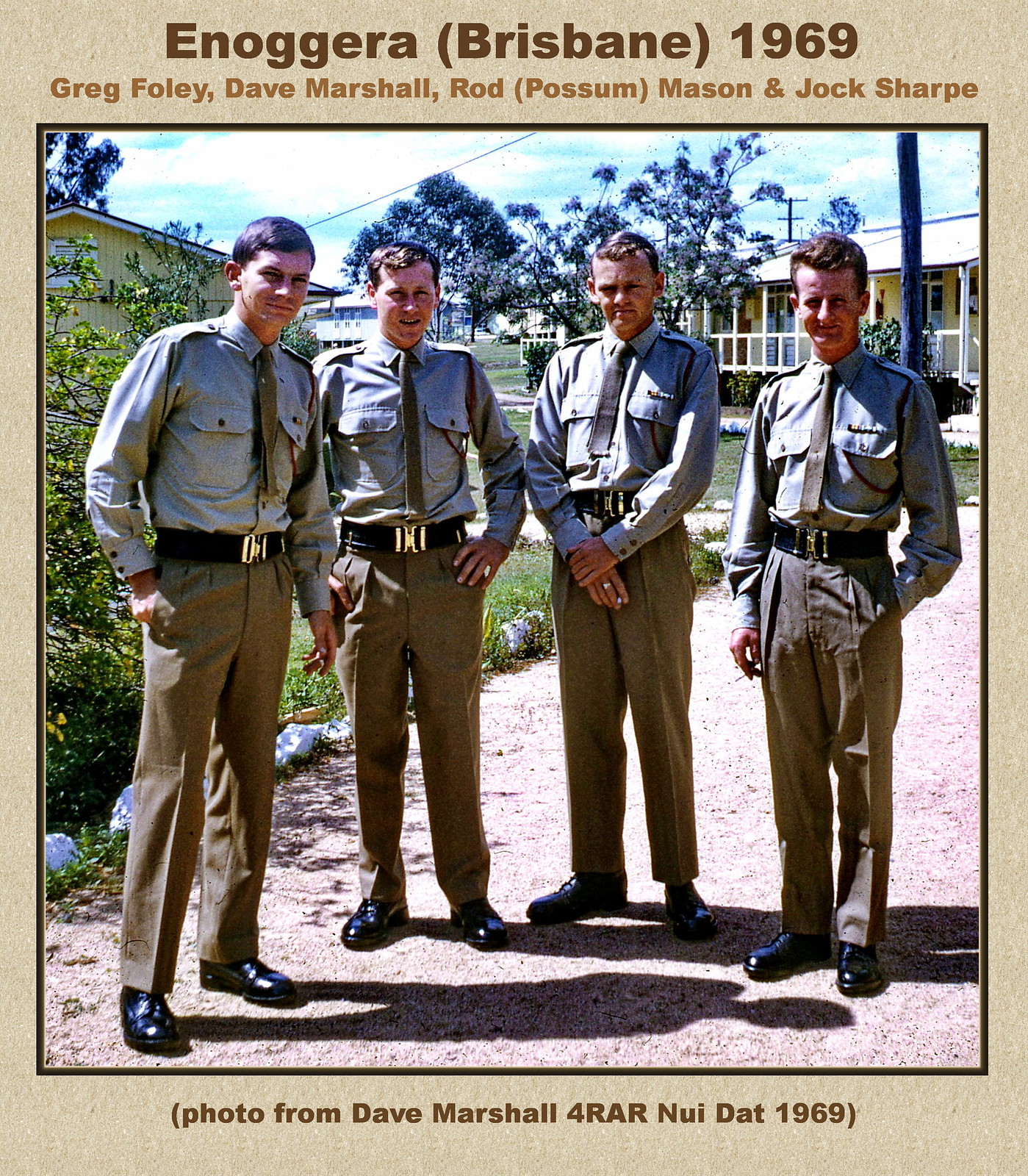This is a tall, rectangular poster framed in textured brown with a darker brown inner frame. The frame is thinner on the sides and thicker at the top and bottom. 

At the top of the poster, in brown font, it reads "Enoggera (Brisbane), 1969." Beneath this, in lighter brown font, the names "Greg Foley, Dave Marshall, Rod (Possum) Mason, and Jack Sharp" are listed. At the bottom, in dark brown font, it notes that the photo is from Dave Marshall for RAR Newey Dot, 1969.

The central image is a square-shaped outdoor scene depicting four young men standing in a row. They are dressed in matching uniforms, which consist of light brown pants, light gray long-sleeved shirts, and thick, dark belts with gold buckles. They also wear black shoes. Behind them, some houses and trees are visible, enhancing the outdoor setting. The men appear to be in some kind of uniformed role, possibly forest rangers or a similar profession.